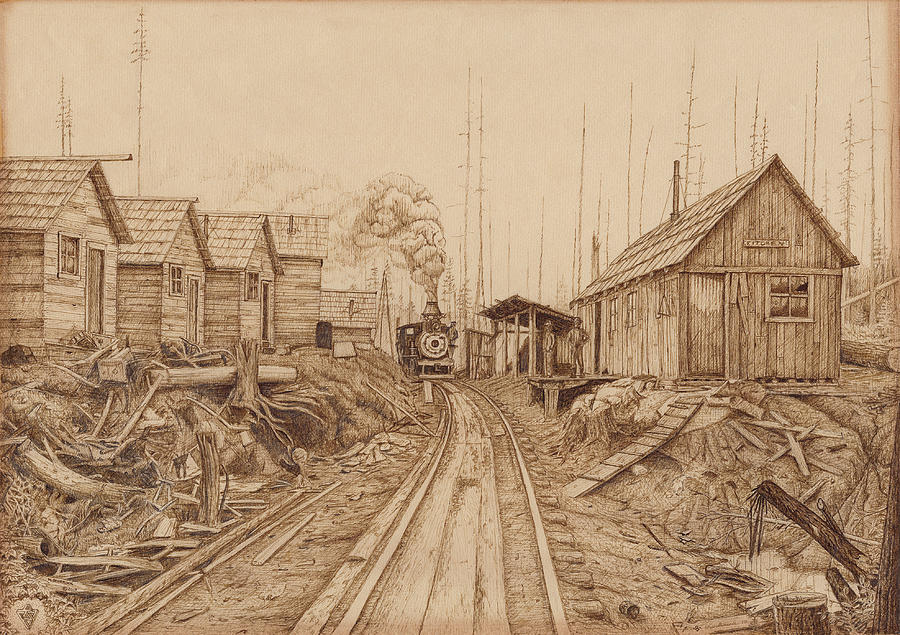The image depicts a detailed drawing based on a historic outdoor scene, rendered in shades of light peach and brown tones. At the center of the image, an old steam engine train travels down a track, emitting steam from its chimney. The front of the train features a prominent circular design. On both sides of the track, a range of small wooden buildings lines the scene. On the left, there are five such structures, surrounded by various debris including branches, wooden planks, and other materials, suggesting recent construction or ongoing work. On the right side, situated near a stable, there is a platform with two drawn figures; one stands on the platform while the other appears near a building marked with a sign that reads "kitchen." The composition's clarity is decent, and despite being monochromatic, it effectively conveys a bright and clear setting through the use of light shading and effective distribution of light and dark areas.